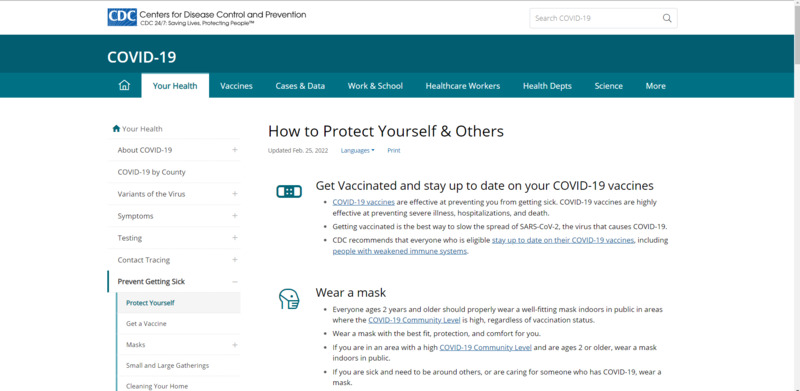The image features a top section with a white border and the CDC (Centers for Disease Control and Prevention) logo. It includes the tagline "CDC 24/7: Saving Lives, Protecting People." Below the logo is a search box labeled "Search COVID-19," followed by a bluish-grayish menu with several options: COVID-19, Your Health, Vaccines, Cases and Data, Work and School, Healthcare Workers, Health Departments, Science, and More. 

Under this menu, there is updated information on how to protect oneself and others, dated February 25, 2023. Various options to change the language or print the page are also available. The main content emphasizes the importance of getting vaccinated and staying up to date with COVID-19 vaccinations, highlighting that COVID-19 vaccines are effective at preventing illness, severe sickness, hospitalization, and death. The CDC strongly recommends vaccination as the best way to slow the spread of SARS-CoV-2, the virus that causes COVID-19, especially for individuals with weakened immune systems.